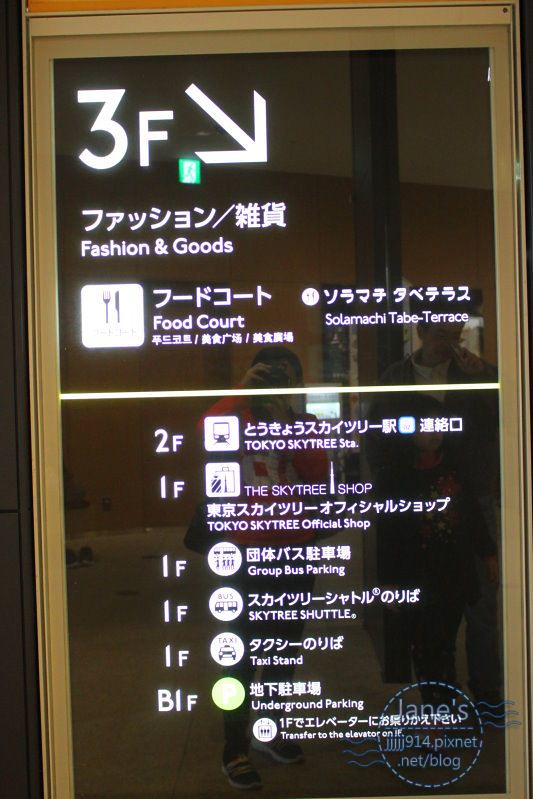This photograph features a reflective window with a medium yellow-brown frame and dark tinted glass. The main focus is a multi-lingual sign displaying both Asian characters, likely Taiwanese or another East Asian script, and English text. At the very top, in white lettering, it reads "3F" accompanied by a diagonal arrow pointing downward to the right. Below this, it says "Fashion and Goods" and features a small white logo of a fork and knife, indicating a food court. The English text also mentions "Sola Mache Tabe Terrace." 

A white horizontal line runs through the middle of the window, below which additional information is listed including:
- "2F" with a small train icon labeled "Tokyo Skytree"
- Various amenities on "1F" such as "The Skytree Shop," "Group Bus Parking," "Skytree Shuttle," and "Taxi Stand"
- "B1F" for "Underground Parking."

The window’s reflective surface shows the faint image of the photographer and possibly other people. At the very bottom of the window, there is a faint logo that reads "janes914.pixnet.net/blog." This sign appears to be an informational guide, likely for a mall or shopping center, providing directional cues and listings for different floors and services.